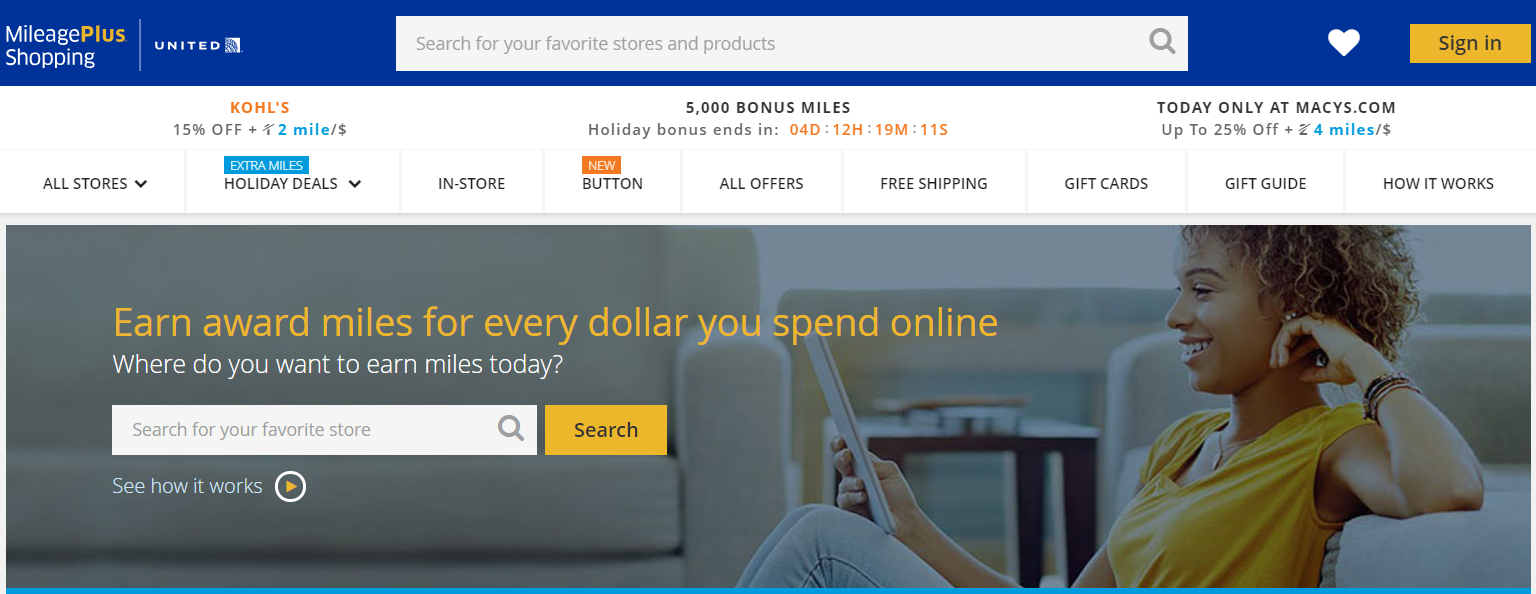Screenshot of the MileagePlus Shopping Website Homepage

At the very top of the webpage, a blue banner displays the text "MileagePlus Shopping" in white, with the word "Plus" highlighted in yellow, followed by the United Airlines logo. Below this, a prominent white rectangular search box invites users to "Search for your favorite stores and products," accompanied by a white heart icon and an orange sign-in button.

Directly beneath the search box is a promotional advertisement boasting "Kohl's: 15% off plus 2 miles/dollar" and "5,000 bonus miles." A countdown timer indicates that the "Holiday bonus ends in 4 days, 12 hours, 19 minutes, 11 seconds." Adjacent to this, another deal highlights "Today only at Macys.com: Up to 25% off plus 4 miles/dollar."

The website features a navigation bar with clickable buttons for "All Stores," "Holiday Deals," "In-Store," "All Offers," "Free Shipping," "Gift Cards," "Gift Guide," and "How It Works." 

Below this navigation bar is a banner showcasing an image of a black lady adorned with bracelets, dressed in a yellow shirt and blue jeans. She is engrossed in what appears to be an iPad. Accompanying her image, the text reads: "Earn award miles for every dollar you spend online. Where do you want to earn miles today?" followed by another search bar for user convenience.